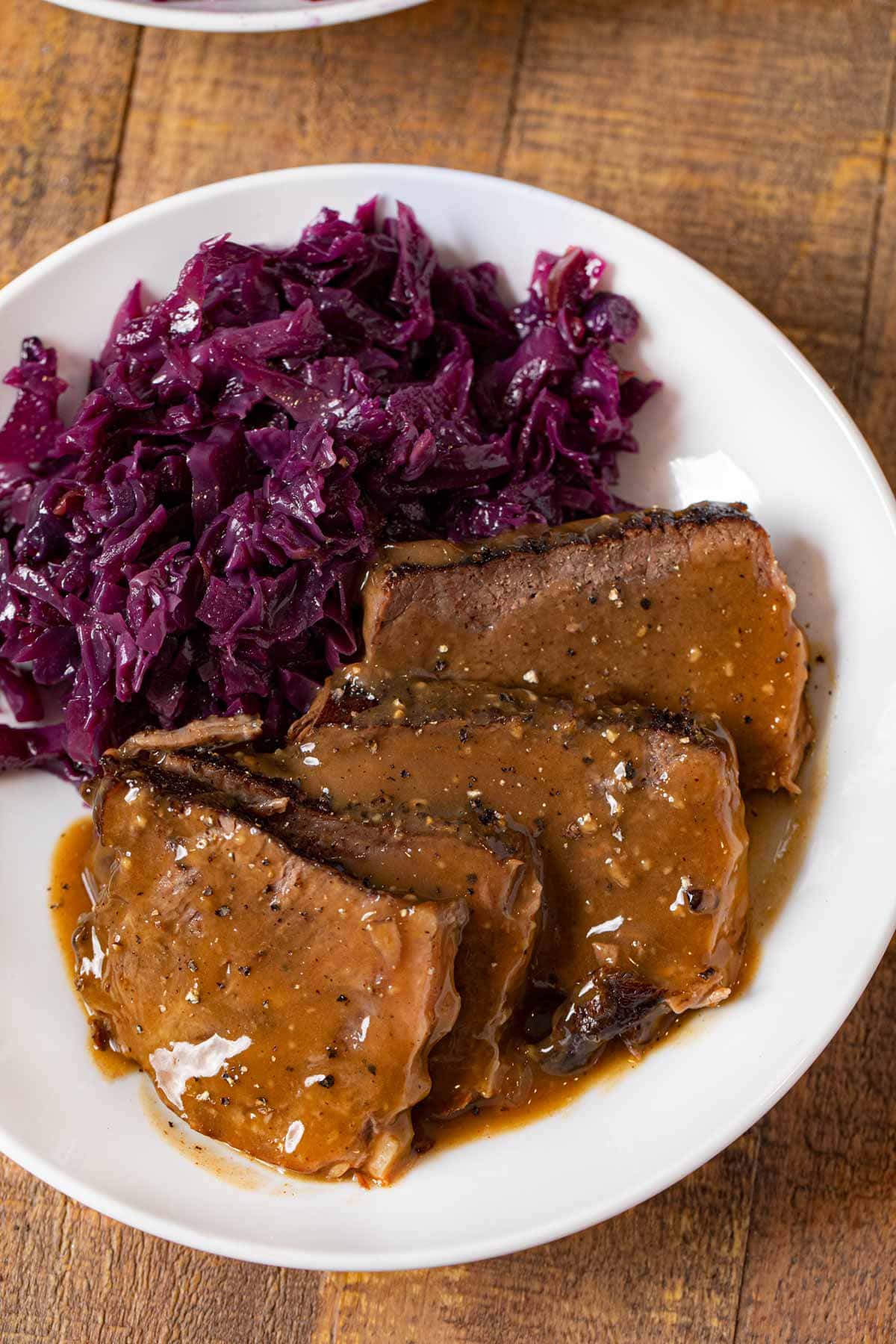The image features a vertical view looking down at a beautifully set wooden table with visible wooden planks underneath. Centered on the rustic table is a white, round ceramic plate. The plate depicts a mouthwatering dish consisting of four slices of beef brisket, arranged diagonally with a shiny, seasoned gravy draped over them. The gravy contains visible chunks of seasoning such as pepper. Adjacent to the meat, occupying the other half of the plate, is a generous serving of deep purple shredded red cabbage. The contrasting textures and colors between the succulent beef and the vibrant cabbage create a visually appealing composition. In the upper left corner of the image, a small glimpse of another plate is visible, hinting at additional culinary delights just out of view.